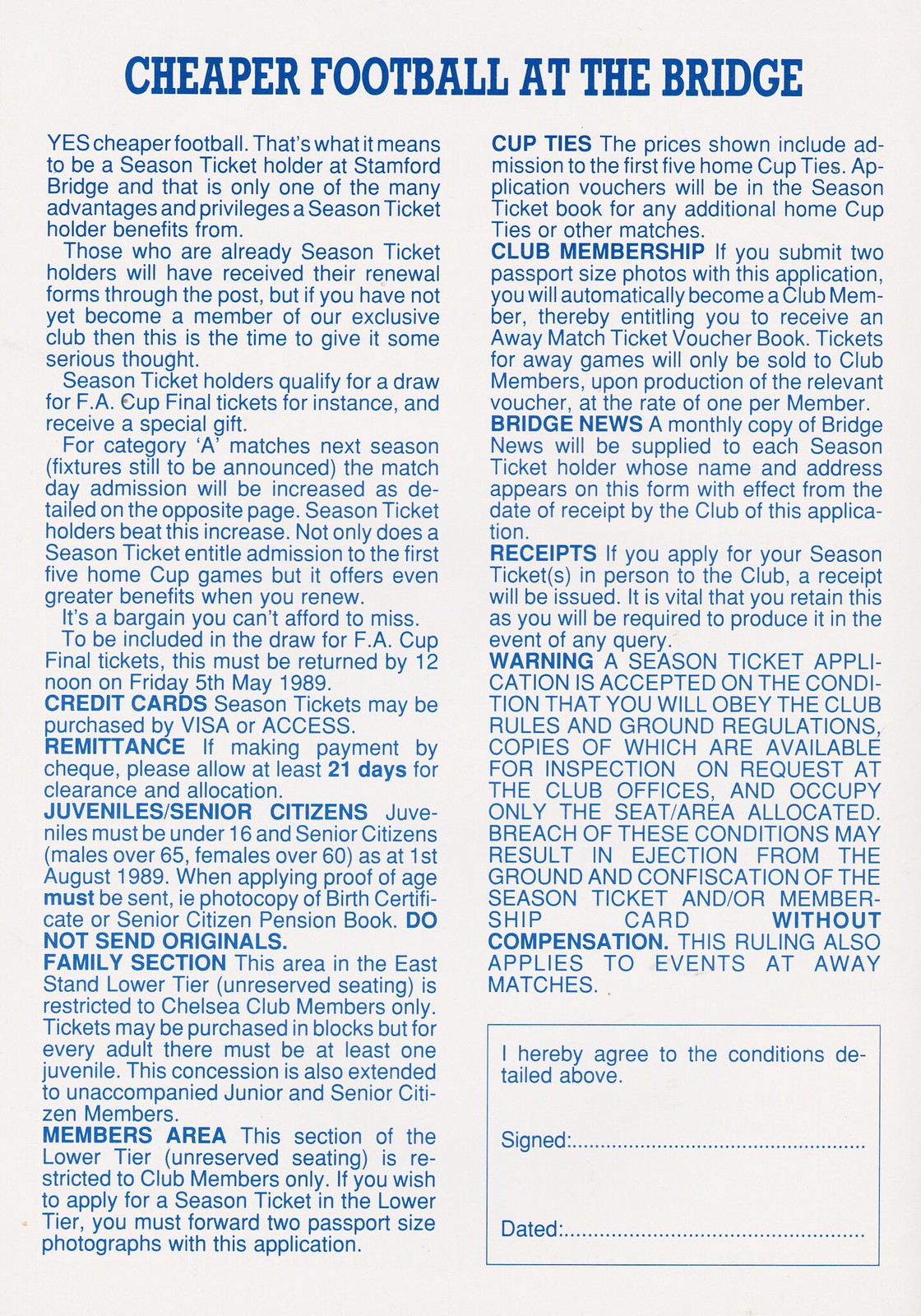The scanned newspaper article titled "Cheaper Football at the Bridge" highlights various advantages and privileges of being a season ticket holder at Stamford Bridge. The article, with blue text on a white background, explains that season ticket holders not only enjoy cheaper football but also many exclusive benefits. It mentions that current season ticket holders should have received renewal forms by post. The article encourages new members to consider joining the exclusive club for perks such as entry into a draw for FA Cup Final tickets, a special gift for Category A matches, and other benefits. 

Season ticket holders can avoid the upcoming match day admission increase and gain admission to the first five home cup ties. To participate in the FA Cup Final tickets draw, forms must be submitted by 12 noon on Friday, May 5, 1989. Payments can be made by Visa or other credit cards, and proof of age is required for juvenile and senior citizens applying for tickets. The family section in the East Stand lower tier offers unreserved seating for Chelsea Club members, with requirements for adult to juvenile ratio for ticket purchases. 

Additional perks include automatic club membership with subsequent access to away match ticket vouchers, and monthly issues of Bridge News. The article concludes with a warning that season ticket applications must comply with the club rules and regulations, with breaches potentially resulting in ejection and confiscation of tickets without compensation. The bottom of the article features a box for applicants to sign, agreeing to the conditions.